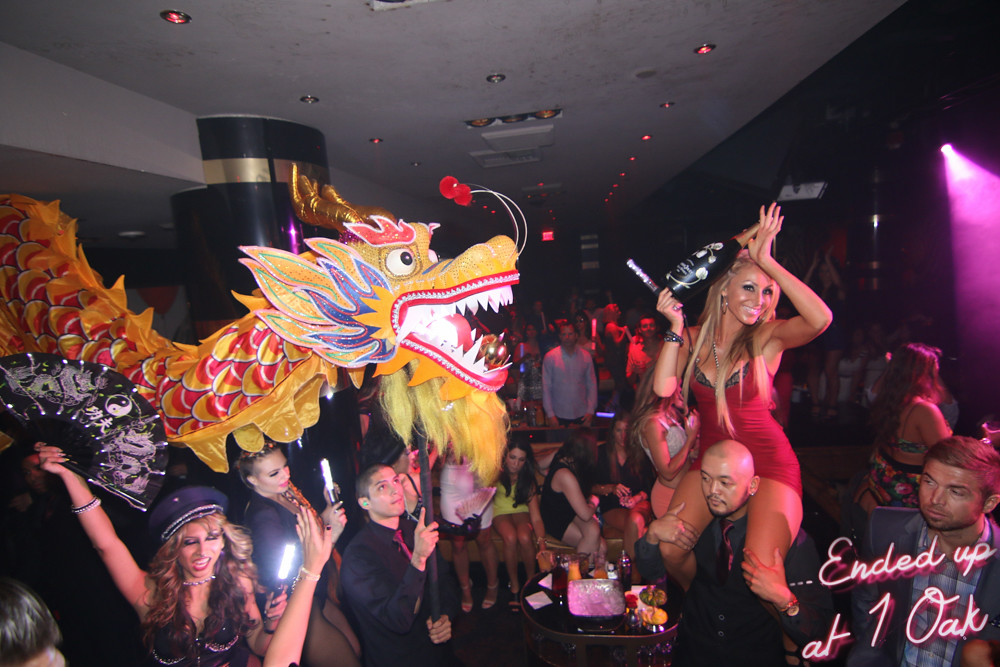The image captures a vibrant scene inside what appears to be a dark nightclub, adorned with pink and red lights that bathe the room in a festive glow. At the center of the excitement, a crowd parades a striking yellow Chinese dragon puppet, its vivid colors and intricate details drawing attention. One of the puppet handlers is a man dressed in black with a red tie, gripping a pole connected to the dragon's head. Off to the right, a woman in a revealing red dress sits triumphantly on a man's shoulders, her long blonde hair cascading down as she raises a bottle of champagne with a jubilant smile. In the foreground, a woman in a sparkly blue outfit, complemented by elaborate makeup and a police officer's hat, waves a black folding fan decorated with yin yang symbols and Chinese characters. The scene is dotted with various people, some mingling and observing, while others lounge on a couch behind a coffee table laden with drinks. The lively atmosphere is punctuated by a neon-style text at the lower right, reading "...ended up at 1OAK."